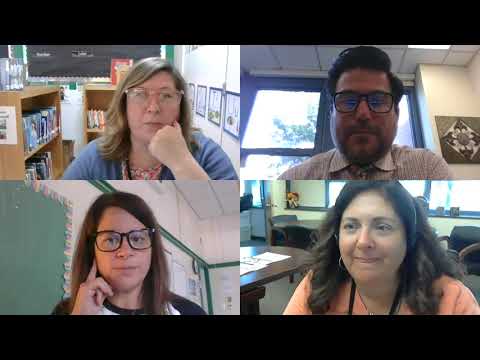In this detailed screenshot of a Zoom video meeting, four individuals are arranged in a quad box display. In the upper left quadrant, a blonde-haired woman with glasses has her chin resting on her fist and is set against a backdrop of bookshelves, unmistakably hinting at an academic environment. The top right panel features a dark-haired man with a beard and dark-framed glasses, seated in front of a window and white wall. He too appears to be in a classroom setting. The bottom left section shows another glasses-wearing woman with long brown hair, positioned in front of a green chalkboard with decorative elements, clad in a black-and-white shirt, with her hand up against her face. Lastly, the lower right quadrant captures a woman with dark hair, wearing a peach-colored shirt, and a visible ID card on a black lanyard. She is set against a background featuring tables and chairs, potentially indicating another academic location. All participants seem to be intently listening, as no one is speaking, adding to the impression that this might be a faculty meeting. The image is framed with black borders at the top and bottom.